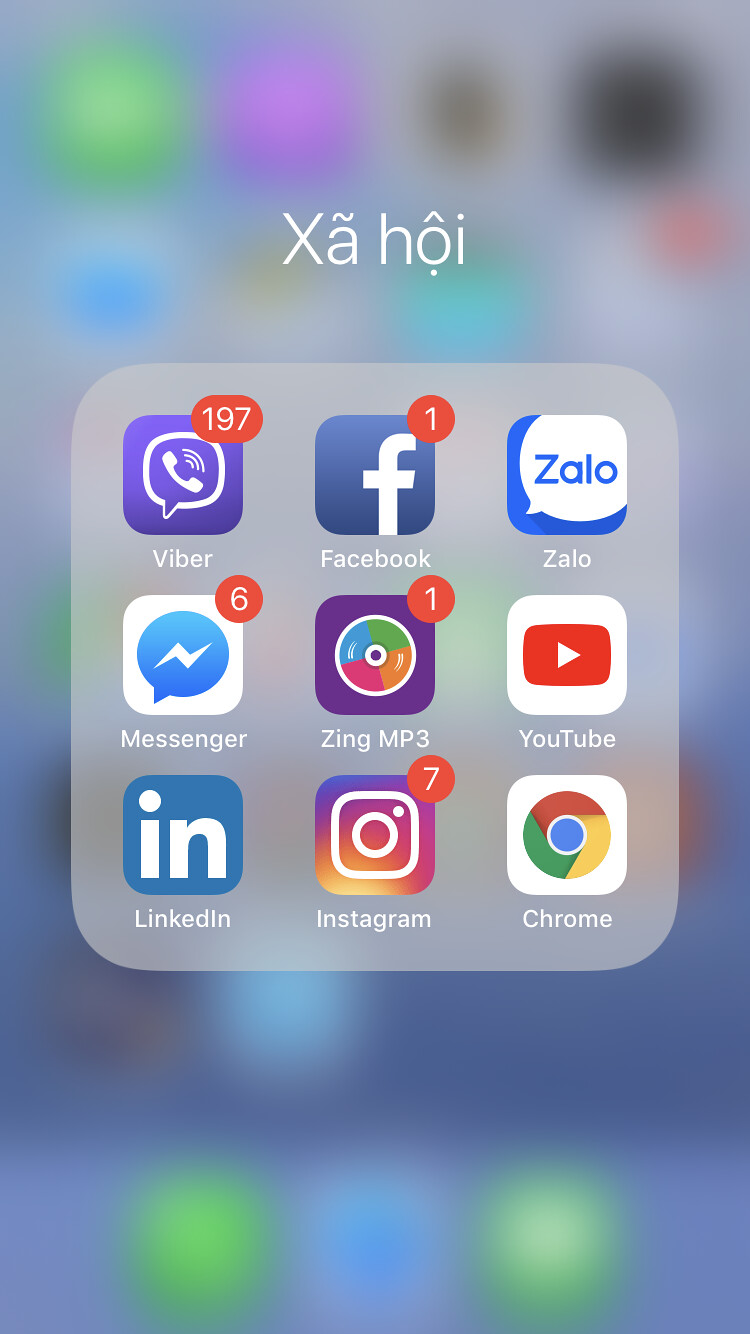The image is a screenshot of an app folder on an iPhone. The background is blurred, focusing on a folder titled with characters resembling "XãHội" - this text includes an 'a' with a tilde, an 'o' with an arrow-like accent above it, and a dot below it, indicating it might be in Vietnamese. Below the folder name is a large gray square divided into nine smaller squares, each representing an app icon. 

Starting from the top left:
1. **Viber**: A purple square with a white speech bubble that contains a phone icon and three lines indicating sound. It shows 197 notifications.
2. **Facebook**: A blue square with a large white 'F' and 1 notification.
3. **Zalo**: A blue square with a white speech bubble containing the word "Zalo" in blue. It has no notifications.

In the second row:
1. **Messenger**: A white square with a blue speech bubble featuring a white lightning bolt. It has 6 notifications.
2. **Zing MP3**: A purple square with a multicolored circle (blue, green, orange, and pink) in the center. It has 1 notification.
3. **YouTube**: A white square with a red rectangle containing a white play button (triangle) in the center. It has no notifications.

In the bottom row:
1. **LinkedIn**: A blue square with the white letters 'in'. It has no notifications.
2. **Instagram**: A square with a rainbow gradient (purple, yellow, orange, pink) background and a white outline of a camera. It has 7 notifications.
3. **Chrome**: A white square with a multicolored circle (red, green, yellow) containing a blue dot in the center. It has no notifications.